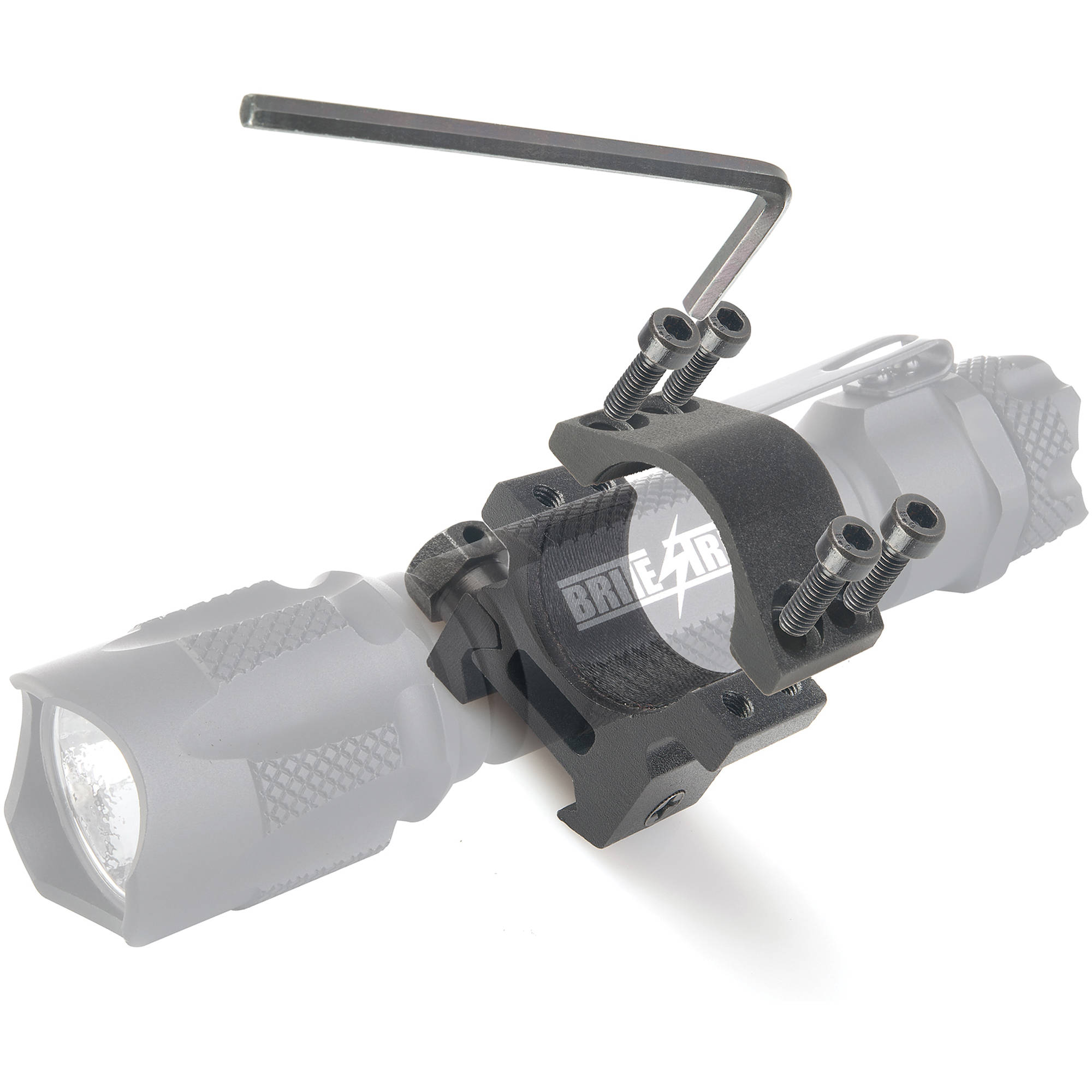This detailed image showcases a device designed to mount a flashlight onto a wall. The primary focus is a sturdy black metal bracket with four heavy-duty screws that secure the flashlight in place. The image is set against an isolated white background, highlighting the functional elements of the device. A ghostly, semi-transparent flashlight is depicted at an angle, from the lower left to the upper right, to illustrate how it fits within the bracket. The flashlight features grip areas near the lens and at the end, displaying faint but legible white lettering that reads "B-R-I-T-E" followed by partially obscured characters. An Allen wrench is positioned above the bracket, implying the method of tightening the screws. The flashlight’s ghostly appearance accentuates the bracket’s design and function, emphasizing how the mounting system would securely hold the flashlight.